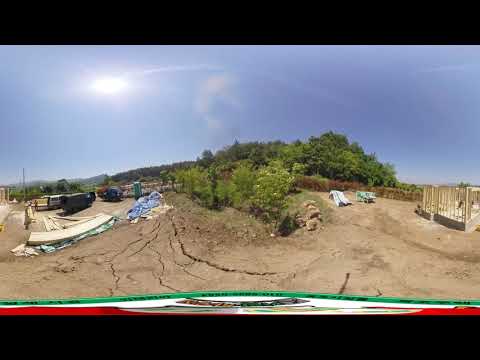In this photograph taken outside, the scene depicts a dusty, dirt-covered plot of land, suggesting an area under construction. In the foreground, brown, cracked earth dominates the landscape with scattered pieces of wood and both blue and green tarps draped on the ground. Various parked vans and vehicles are visible, presumably belonging to the construction workers present at the site.

On the right side of the image, the wooden frame and foundation of a house under construction are visible, hinting at ongoing building activities. Adjacent to this structure, a few stacks of building materials are organized neatly along with a nearby wooden gate.

The background showcases a sandy area transitioning into a grassy field dotted with bushes, leading up to a distant hill blanketed with a dense collection of green trees. The sky overhead is clear and vibrant blue, featuring just a few wispy clouds, and the bright sunlight bathes the entire landscape, creating stark contrasts and clear, vivid details.